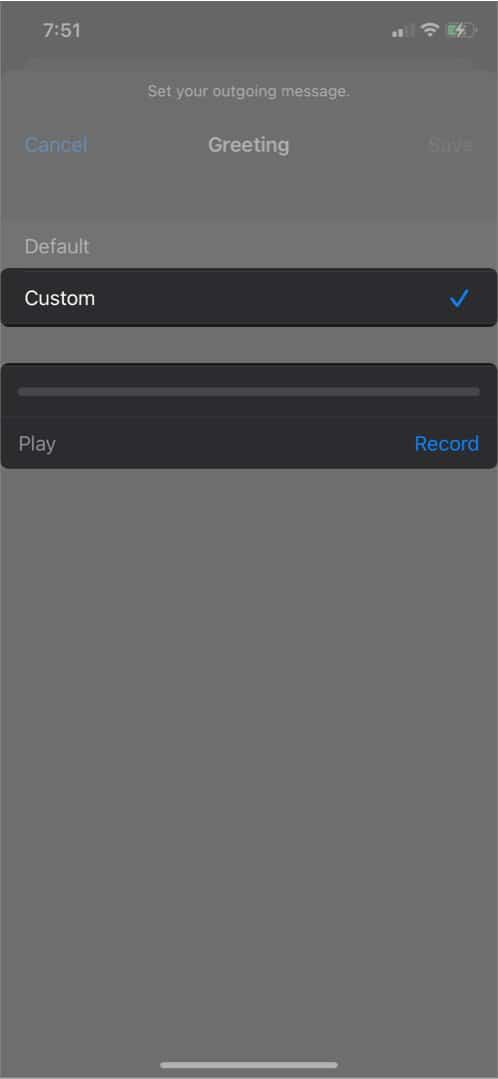The image depicts a cell phone screen with a gray background. At the top of the screen, standard cell phone icons are visible: the time displayed at 7:51 on the top left, followed by a signal connection icon, a Wi-Fi icon, and a half-full battery icon that is part green and part gray on the top right. Below these icons, light gray text reads, "Set your outgoing message."

Further down, the text "Greetings" appears, accompanied by a blue "Cancel" button on the left. Below this are two options: "Default" and "Custom", with "Custom" selected and highlighted in black. The word "Custom" is white and has a blue checkmark on the right-hand side.

Approximately 60% of the way down the image, there is a black option bar featuring the text "Play" on the left and "Record" on the right in blue. The remaining bottom portion of the screen displays a gray background with a single light gray bar centered at the bottom.

The screen is presented as part of a tutorial by Sam, who thanks the viewers and signs off at the end with, "Thanks for watching. I'm Sam. I'll see you in the next video."